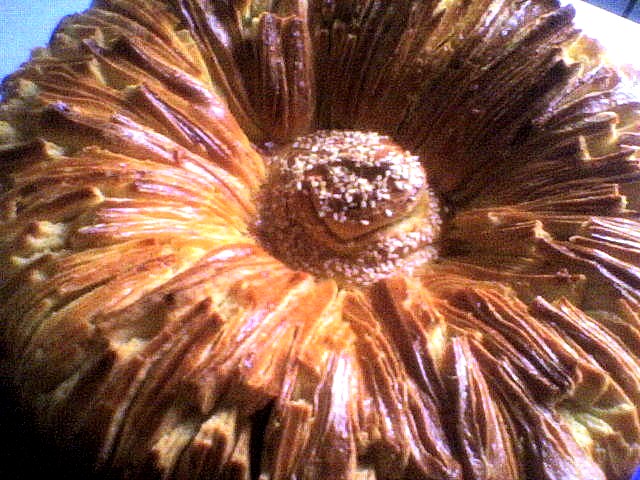The image features a detailed close-up of a circular flower that intriguingly resembles a baked good due to its varied shades of yellows, browns, and tans. The flower is covered in numerous small pebbles radiating from the center, which includes semi-organized white dots that spiral outwards, slightly becoming larger towards the center. These white spots are likely pollen. The flower's petals exhibit a gradient from yellow to brown, extending outward to form a ring of numerous petals. The flower rests on a white table, with light illuminating it from a 45-degree angle on the right, casting shadows across its intricate surface. In the background, the setting includes a mix of blue, possibly a sky or mottled surface, along with hints of nearby furniture such as another table leg in the upper right corner. The composition is heavily focused on the flower, occupying most of the frame, with the image taken from an overhead angle.